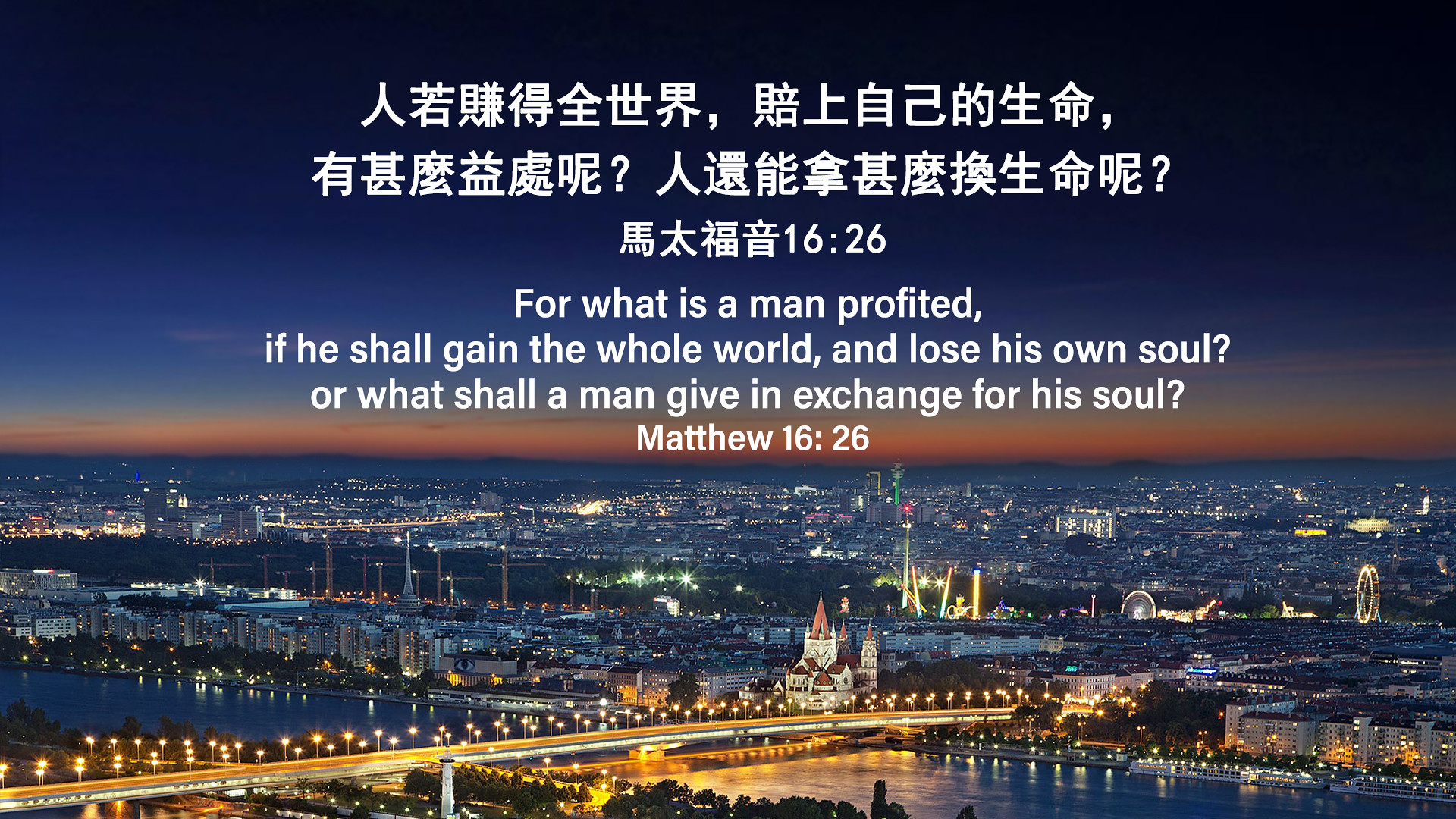The image features a sprawling cityscape viewed from a distance, with the last vestiges of sunset casting an orange-brown hue on the horizon that gradually transitions to a deep blue, eventually becoming almost black at the top. The city is densely packed with numerous buildings and twinkling lights, creating a mesmerizing urban jungle. In the foreground, a long bridge adorned with yellow streetlights stretches across a waterway, reflecting beautifully off the water.

At the top of the image, an inspirational quote is written in Chinese characters, with its English translation located below. The English text reads: "For what is a man profited, if he shall gain the whole world and lose his own soul? Or what shall a man give in exchange for his soul?" - Matthew 16:26. This poignant message adds a layer of depth to the stunning visual, juxtaposing the allure of the illuminated city with a profound reflection on spiritual well-being.